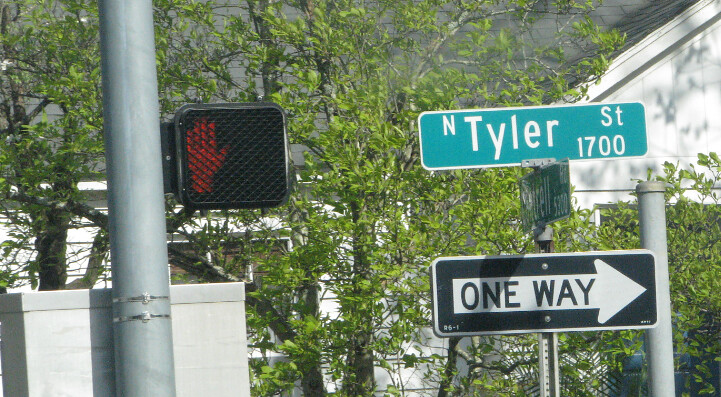The image depicts a detailed urban intersection scene prominently featuring various street signs and signals. In the foreground, there is a large grey pole with a thick, square grey box attached to it via clamp bands. To the right of this pole is a "don't walk" sign fashioned from a black mesh, displaying a red hand. Adjacent to the walking sign, another grey pole supports a collection of street signs. At the top, a green sign with a teal blue background and white outline reads "N Tyler Street 1700." Below it, a one-way sign, featuring a white outline, black background, and a white arrow pointing right with black letters saying "one way," is visible. In the background, a white house with a steep grey roof stands, partially obscured by at least one large tree or hedge. This intersection scene is framed by lush greenery, including multiple trees and bushes with vibrant green leaves.